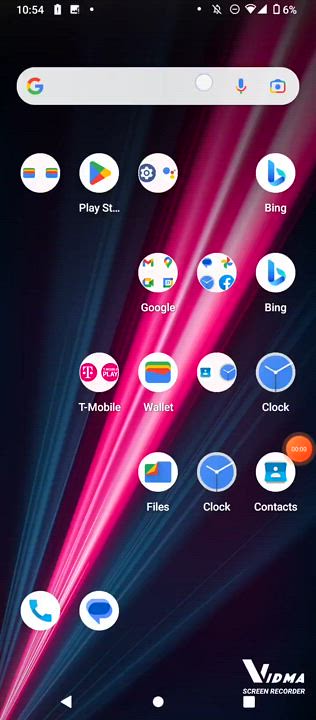The image is a screenshot of a cell phone screen with a vertical portrait orientation. The background image features a black backdrop adorned with a series of blue streaks that emanate from the bottom left corner and spread upwards towards the top right. At the center of these blue streaks is a prominent pink streak, interwoven with pink, red, and white highlights, creating a striking beam effect.

At the top of the screenshot, the phone's status indicators are visible, displaying the time as 10:54 in the top left corner and the battery level at 6% in the top right. Below these indicators, there is a Google search bar, featuring the Google logo on the left and a microphone and picture symbol on the right.

The app screen below the search bar shows several app icons arranged in a grid. The visible apps include Google Play Store, T-Mobile, Wallet, Files, Clock, Contacts, a duplicate Clock icon, and two Bing icons. At the bottom left corner of the screen, there are phone and chat symbols, while the bottom right corner displays the Vidma Screen Recorder logo. The navigation bar at the very bottom of the screenshot contains the standard triangle, circle, and square buttons.